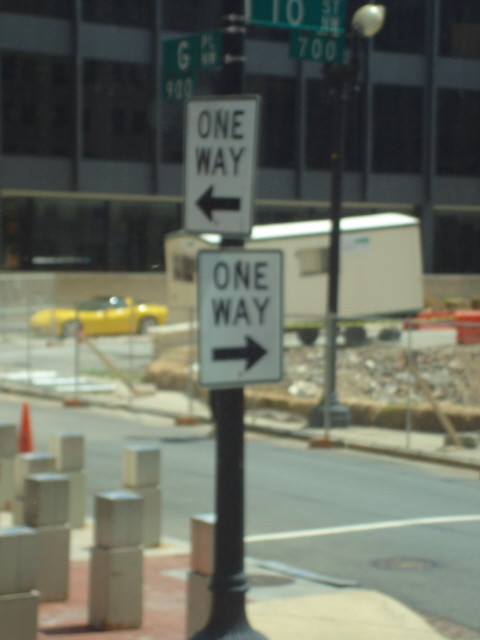The photograph, though slightly unfocused, captures a dynamic urban street corner from a slightly elevated perspective. At the forefront, a paved road intersects with a cement-block sidewalk, guiding viewers' eyes to the central subject of the image: a tall, black pole. Mounted on the pole are two one-way signs with contrasting arrows, one pointing right and the other left, highlighting the city's navigational aids. Atop these signs, three green street markers inform the viewer of the location: "G," "10," and "700." Behind the pole, a construction site bordered by a fence contains scattered mounds of dirt, signaling ongoing development. In the midst of the construction's bustle, a striking yellow sports car stands out, parked just behind the fenced area. Towering in the background, sleek skyscrapers loom over the scene, completing the cityscape.